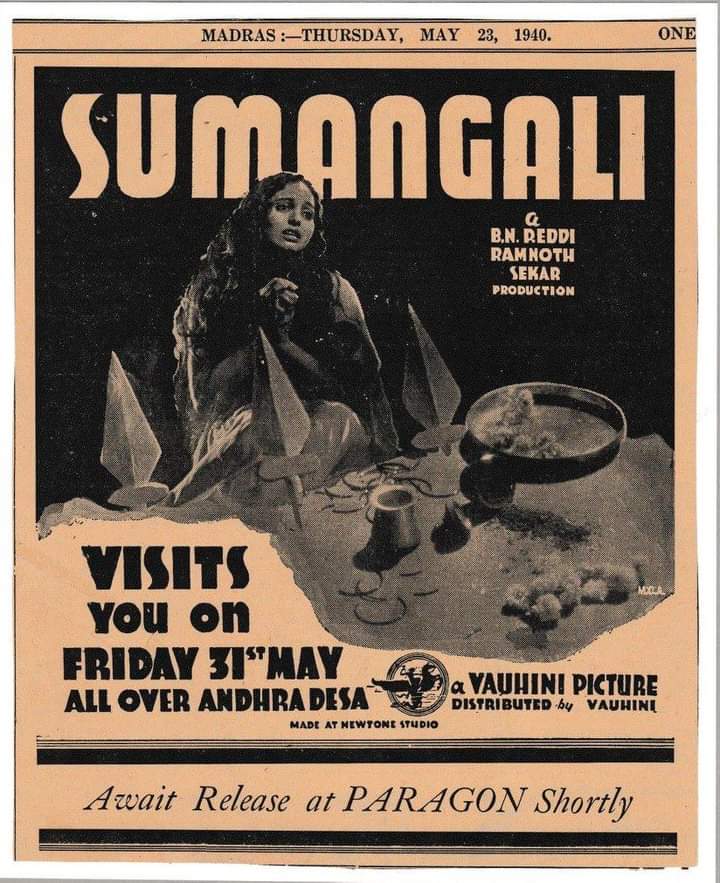This sepia-toned image, scanned from an old newspaper or flyer from Madras dated Thursday, May 23, 1940, promotes a production titled "Sumangali." The central focus is a female figure, possibly an actress, dressed in a traditional gown with her hands folded, perhaps in a gesture of greeting or prayer. The text mentions multiple names, including BN Ready, Ramnath, and Zakhar Production, suggesting key figures involved in the making of "Sumangali." It intriguingly announces, "Visits You on Friday, 31st May, all over Andhra Desa," indicating a widespread release. At the bottom, it's noted that the production is a Vahini Picture, "Made at New Tone Studio," and will be "Distributed by Vahini," culminating with a call to "Await Release at Paragon Shortly." Adding to the vintage feel, a logo features a winged horse or unicorn. The ad, with its historical context and graphical details, exists as a captivating artifact from 1940s Indian cinema.